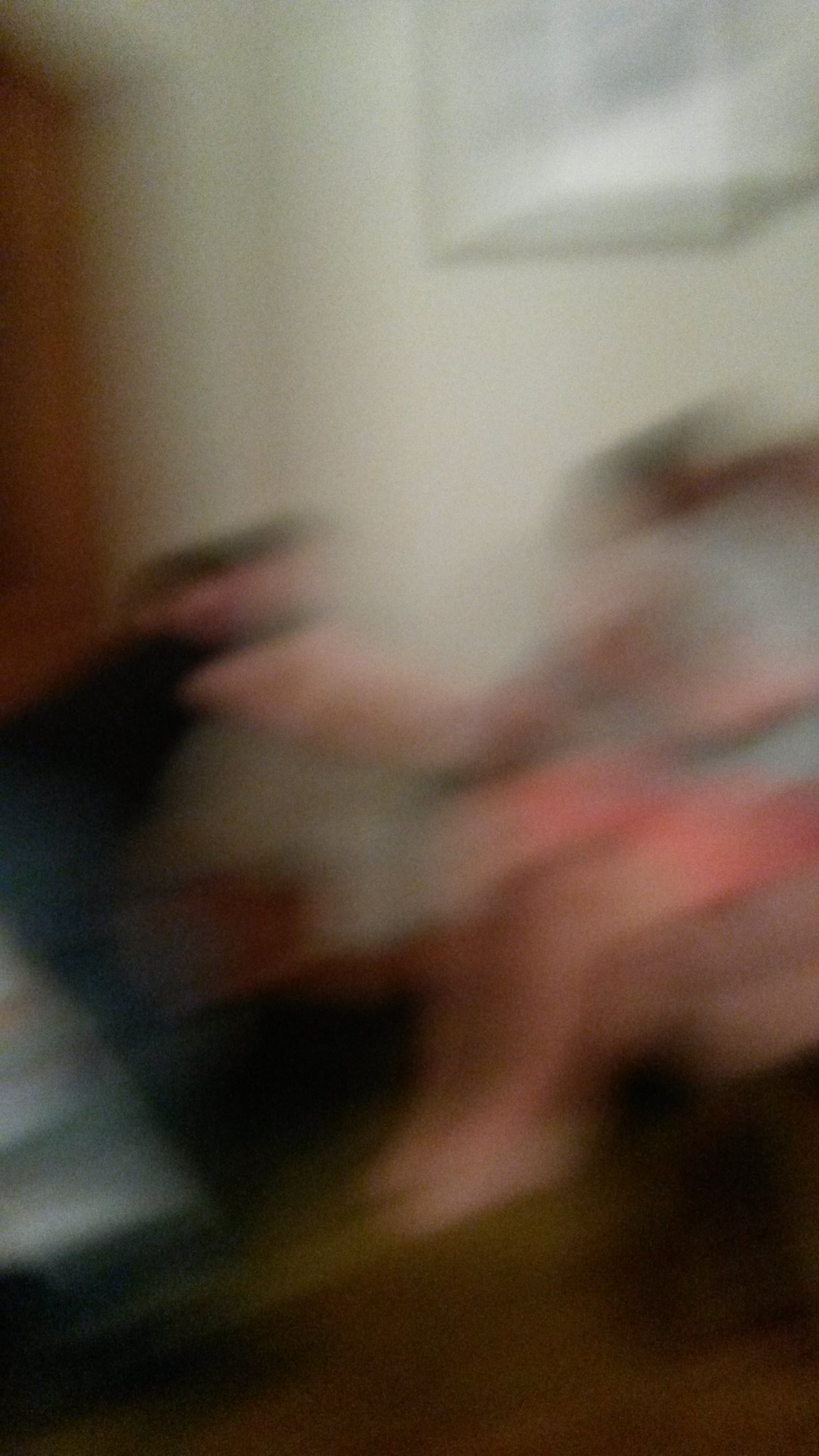In this slightly blurred image, you can discern two individuals. The first person is seated in a chair, donning a gray top adorned with a red design on the front. They are also wearing coral pink shorts. Their dark brown hair appears to be either tied back or cut short. The second person is kneeling beside the chair, extending their arm towards the seated individual. This person is dressed in a black shirt, with their entire right arm and the right side of their face visible, although somewhat obscured by the blurriness of the picture.